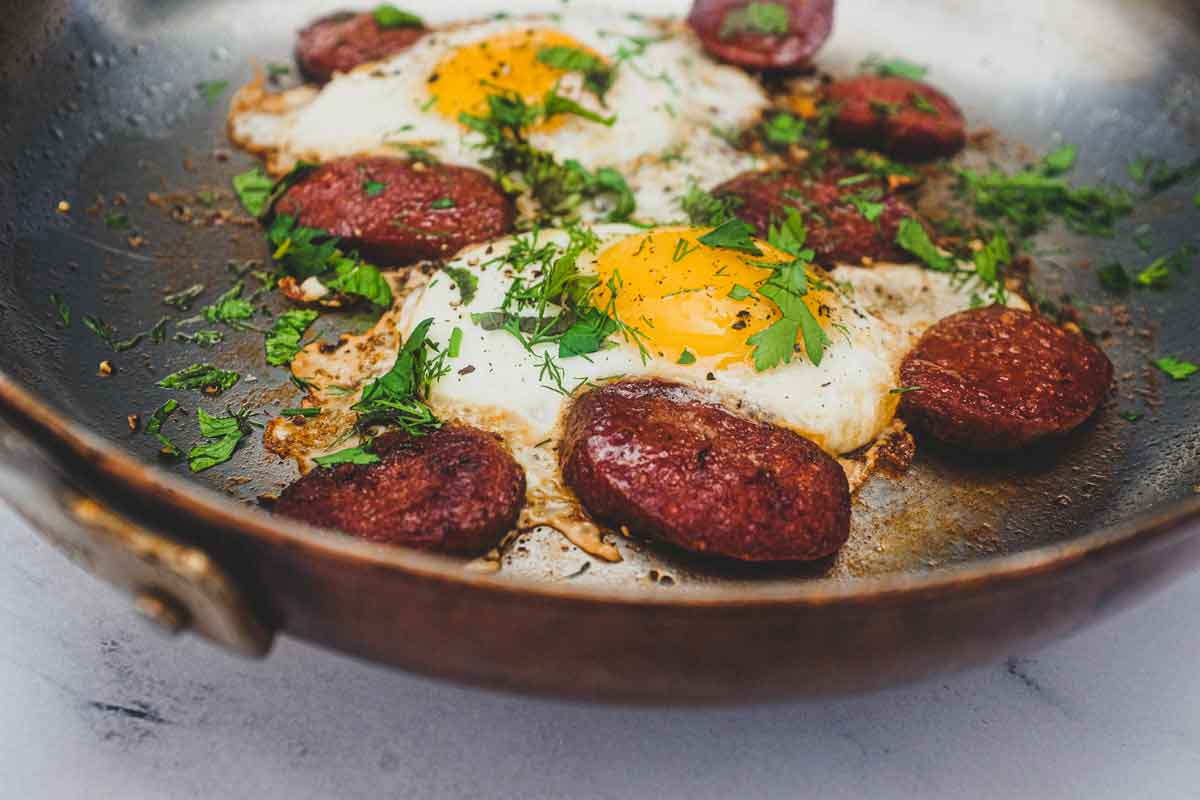This detailed photograph captures a close-up view of a rustic frying pan filled with a delicious-looking meal. The pan, which appears to have a well-used and well-loved cast-iron look with a metal interior and a rivet on the side, is slightly blurry at the bottom edge of the image. The close-up nature of the photo emphasizes the food within the pan, which consists of two sunny side up eggs, their white edges contrasting with rich yellow yolks. The eggs are garnished with green parsley flakes, adding a vibrant touch. Surrounding the eggs are pieces of dark red sausage, circular and oval in shape, complementing the dish with their nicely browned, greasy appearance. There's also a hint of oil and browning around the food, enhancing the appeal of the cooked meal. The background of the image transitions from light gray at the top corners to a darker gray towards the center and bottom edges, highlighting the rustic brown edge of the frying pan.